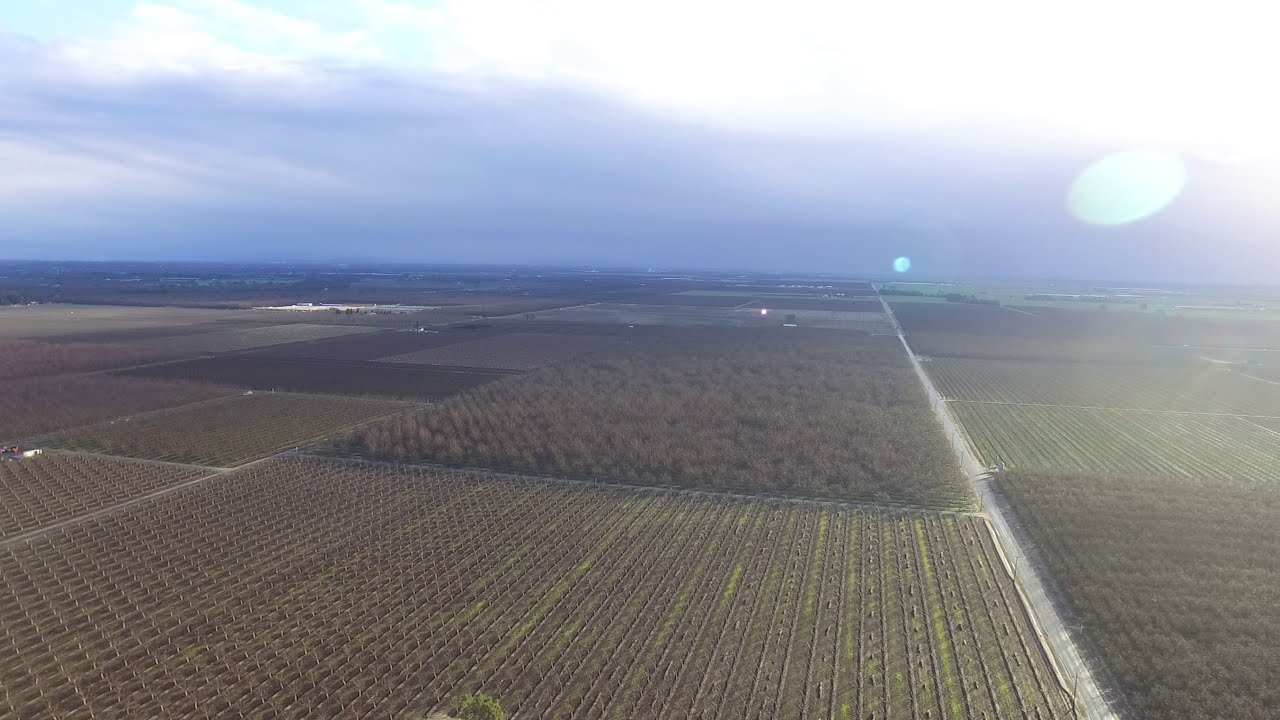The image showcases an aerial view of a rural landscape, featuring a patchwork of farm fields, a strip of road, and a cloudy sky. The bottom portion of the image is dominated by approximately 8 or 9 sections of farmland, characterized by varying shades of brown and green. Some crops appear taller and bushier, particularly in the middle and to the right of the image, while other sections are flatter and darker in color.

On the right side of the image runs a road, extending vertically halfway up before disappearing. The left side and the central part of the image are filled with additional farm fields and clusters of trees. The top third of the image reveals an overcast sky with predominantly white and light blue clouds. The sun is faintly visible in the top right corner, appearing as a pale white spot due to the cloudy conditions. Notably, there are a couple of bright reflections near the right side, likely from the camera lens.

This serene, midday scene captures the essence of the countryside, devoid of any people, vehicles, or text.